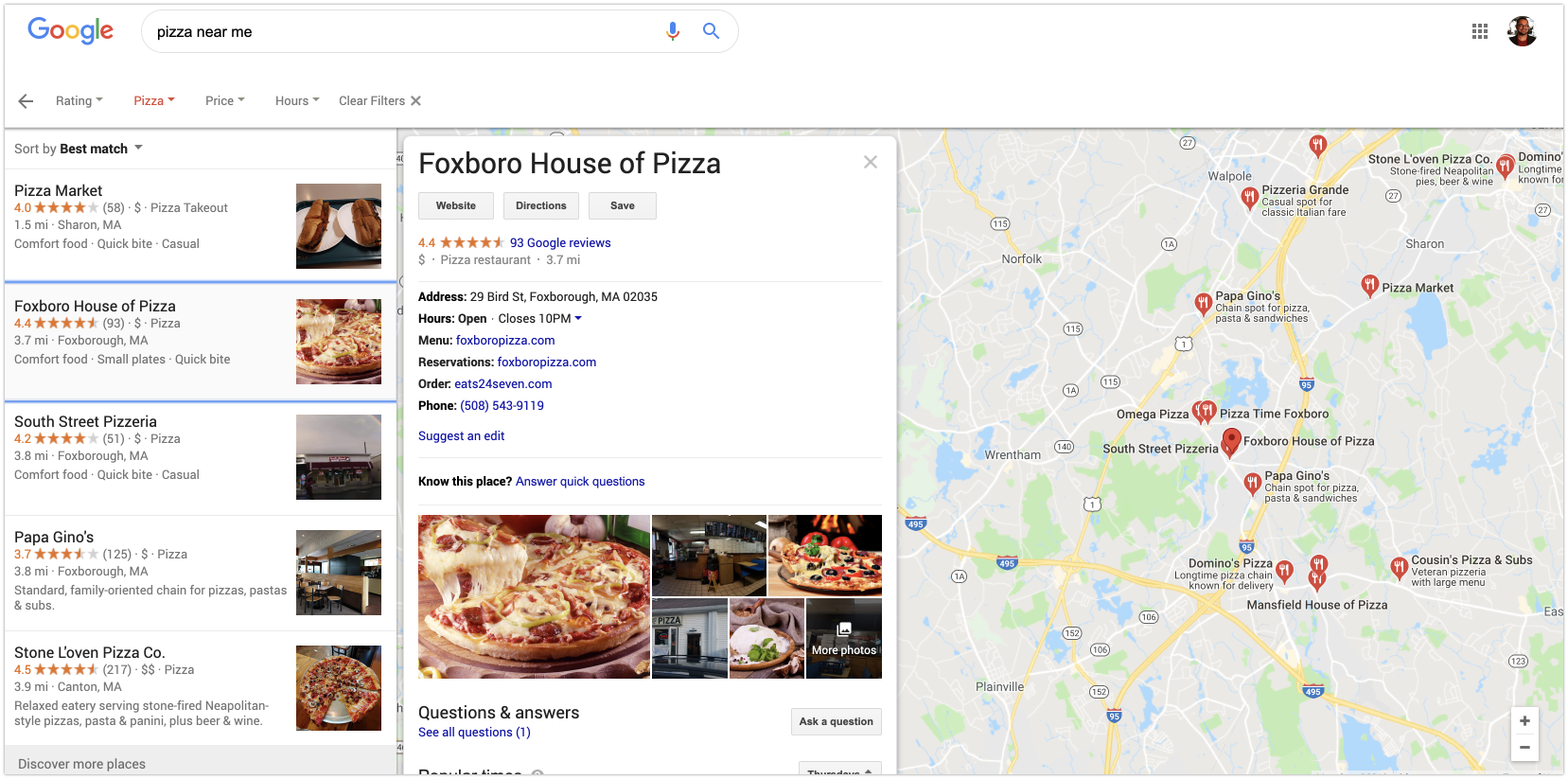A landscape-oriented screenshot of Google Maps search results for "pizza near me" is displayed. The image, approximately twice as long as it is tall, features a thin gray border around its edges. In the upper left corner, the multicolored Google logo (green 'G', red 'O', yellow 'O', blue 'G', green 'L', red 'E') is clearly visible. Below the logo, a white search bar contains the text "pizza near me" in black font, alongside a microphone icon and a magnifying glass icon to indicate options for voice and text search. 

On the right side of the search bar, a circular avatar, likely representing a user profile (potentially female), is positioned. Directly beneath the search bar, navigation options include categories marked by a back arrow and labels such as "rating," "pizza" highlighted in red, "price," and "hours," both with drop-down menus, and a "clear filters" option marked by an 'X'. 

The main content area lists pizza places sorted by best match, including: Pizza Market, Foxboro House of Pizza, South Street Pizzeria, Papa Gino's, and Stone Loving Pizza Company. Foxboro House of Pizza is prominently highlighted, featuring detailed information like address, business hours, menu options, and photos in a large portrait-oriented box. To the right of the results, a map provides a visual representation of the location of Foxboro House of Pizza in relation to its surroundings.